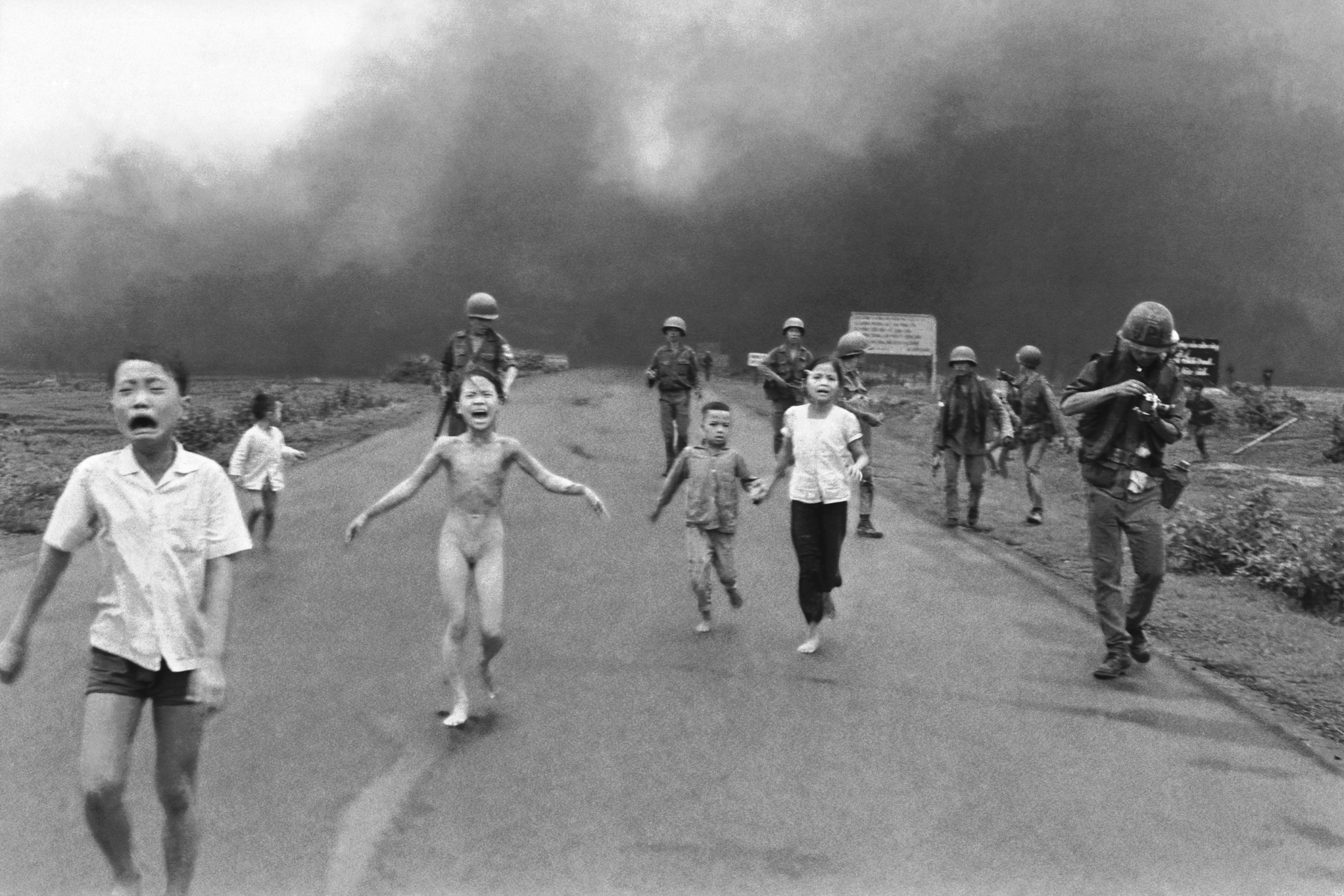This black and white image, likely from the Vietnam War, captures a deeply distressing scene involving a group of horrified children being escorted down a road by armed soldiers. In the center, a completely naked child stands with arms wide open, appearing to cry. To the left of this child, a boy in a white collared shirt and very small shorts looks visibly upset. To the right of the naked child, a young girl and boy hold hands, evoking a sense of shared fear and solidarity. In the background, a dark, ominous cloud of smoke, possibly from a fire, billows into the sky, adding to the dramatic intensity. The soldiers, clad in military gear with hard helmets and weapons, seem to be overseeing or directing the children. One soldier on the right appears to be lighting a cigarette. The entire scene is set against a slightly grassy area bordered by the road, completing this haunting portrayal of the chaos and fear experienced during wartime.